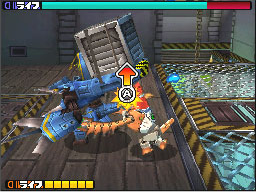The image is a still from a video game depicting an intense battle between two distinctive characters on a wooden platform, likely within a dynamic and colorful environment. The primary characters include a tiger-like figure adorned in brown and yellow stripes with a colorful head and suit of armor, and a blue-hued, horse-like robotic creature equipped with mechanical arms. The robotic creature is holding a large silver box with straps. The two characters are engaged in a fierce wrestling match, amidst a visually vibrant and detailed setting. At the top of the screen, a health bar stretches across, primarily green transitioning to red towards the right, with the number 517 visible both at the top and bottom. A large "POW" symbol with a circle featuring the letter "A" and an upward-pointing arrow takes center stage as they punch each other. The platform itself is surrounded by black and yellow striped caution tape, beneath which lies a gridded area reminiscent of a warehouse floor. Additionally, there are several yellow squares and grills on the right-hand side, potentially indicating a fluid or water below, further adding to the dynamic scene.